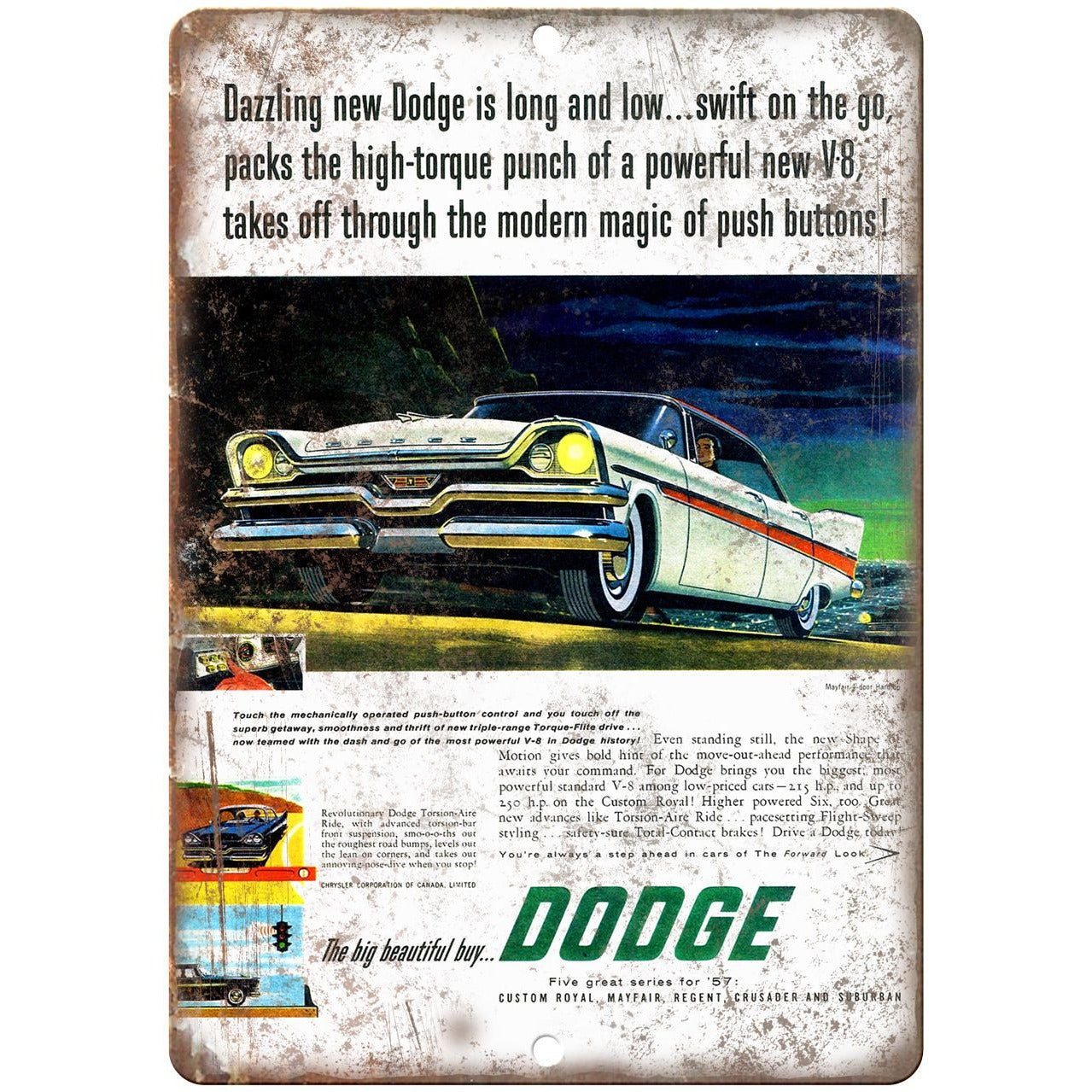This image is a vintage advertisement painted on an aged metal panel, showing significant wear and tear with rust around the edges and peeling paint. At the center of this advertisement, there's a detailed illustration of a classic white Dodge automobile with a red stripe running across the middle and bright yellow headlights. The car features a distinctive chrome grille and two headlights. Above the car, the caption reads: “Dazzling new Dodge is long and low, swift on the go, packs the high torque punch of a powerful new V8, takes off through the modern magic of push buttons.” Below this central image, the ad provides further information about Dodge, showcasing additional smaller images of Dodge vehicles in blue and black, and details about five great series: Custom Royal, Mayfair, Regent, Crusader, and Suburban. The text also emphasizes the tagline "the big beautiful buy" in large green letters, highlighting the affordably priced series for $57. The Dodge symbol is visible in the lower right corner, reinforcing the brand's identity.